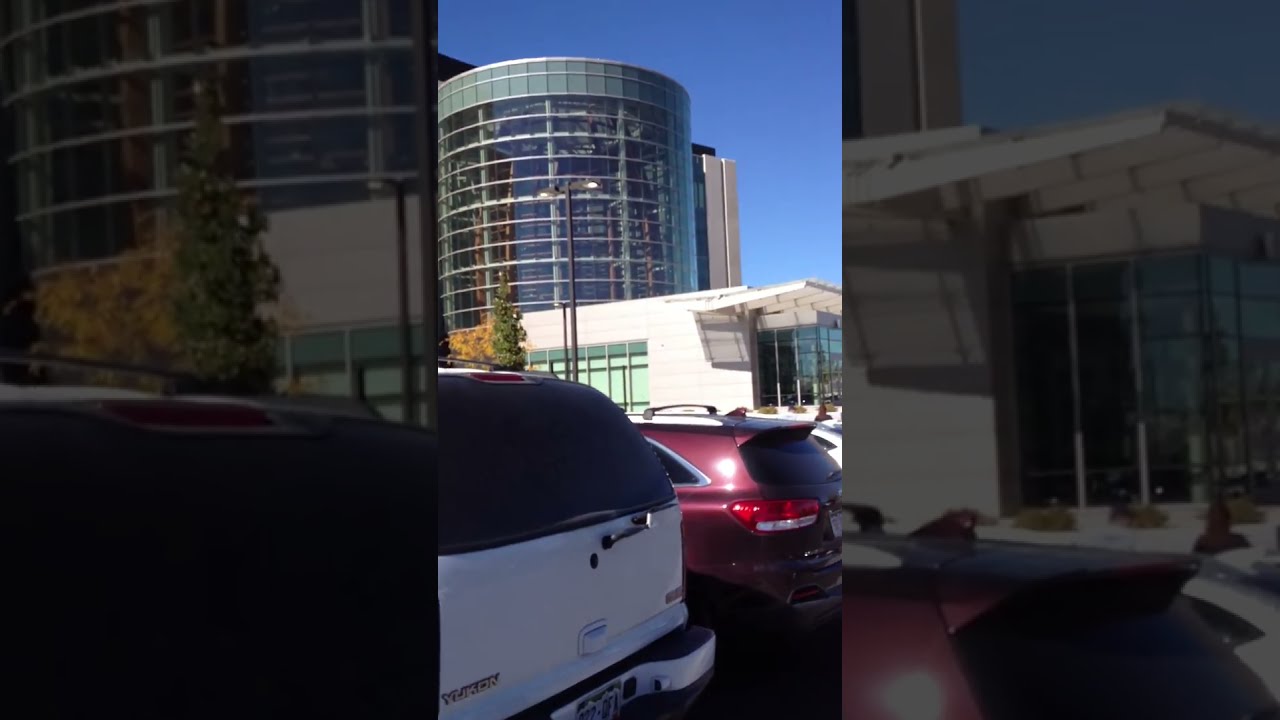The image captures an outdoor parking lot adjacent to an office building characterized by many vertical, glass windows. A variety of vehicles are parked in the lot, with a silver Chrysler SUV prominently positioned on the left. This SUV features a distinct striped grille and a piece of paper inside the windshield. Alongside it, a white SUV with tinted windows is visible. In the background, there are several other parked cars, including red, white, and silver ones. 

A small tree, approximately 10 feet tall, stands near the curb next to the silver SUV, while another, more slender tree with some brown leaves is seen near the building. The parking lot is delineated by white lines on the ground, and the sunny weather casts bright light across the scene. The lower portion of the office building features a black barrier and large, long windows, with circular semi-arches marking some sections. Altogether, the picture presents a typical urban parking lot with cars, trees, and a modern office building in the background.